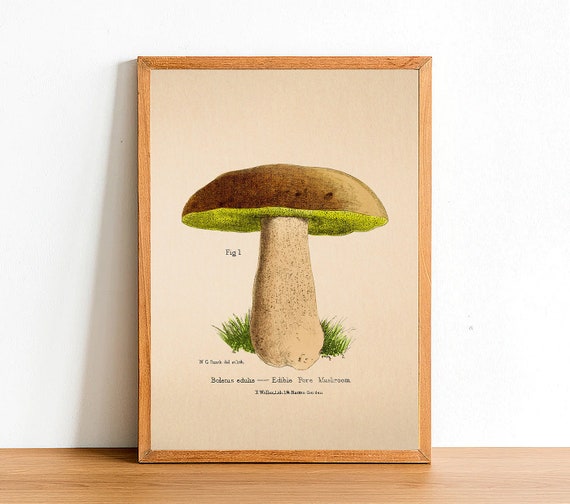The image depicts a framed diagram of a mushroom, with the frame having a thin light tan border. The frame rests against a white wall on a light tan wooden shelf. The mushroom illustration features a dark brown cap with a green underside, supported by a light beige stem. At the base of the stem, a small patch of green grass is visible. To the left of the mushroom, the text "F-I-G-1" can be clearly seen, and at the bottom, partially legible cursive text includes the words "edible pure mushroom."